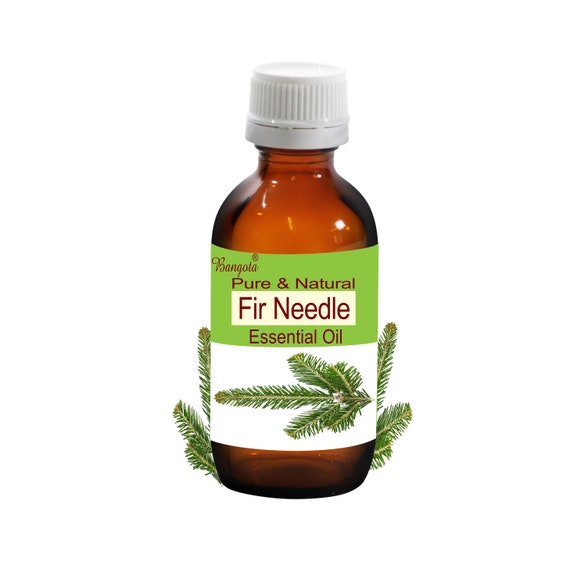This image features a small amber bottle with a sealed white cap, set against a solid white background. The bottle has a label that is green on the top half and white on the bottom half. The top part of the label displays the brand name "Bengola" in cursive print, followed by the words "pure and natural" in standard print. Below this, in a white box, it says "fur needle." Underneath this box, in standard print against the green background, it reads "essential oil." Additionally, the white part of the label features a depiction of a green fir leaf turned to the left side. The image also includes green fir leaves protruding from behind both sides of the bottle.